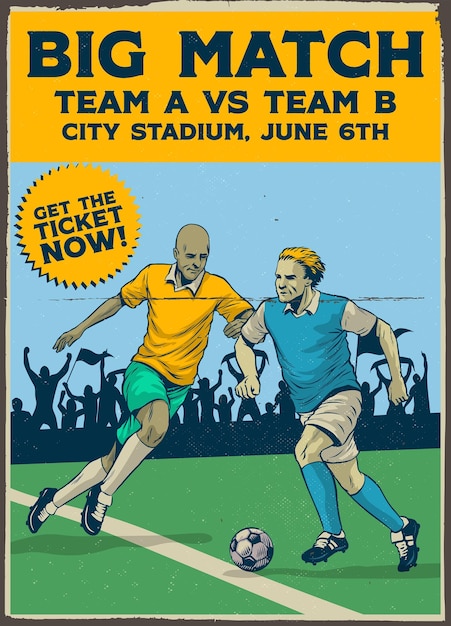This vintage advertisement from the 1930s or 1940s promotes an exciting soccer match between Team A and Team B at City Stadium on June 6th. The ad features bold black lettering at the top that reads, "Big Match, Team A versus Team B, City Stadium, June 6th. Get the Ticket Now." The background of the text is a striking yellow, while the lettering is in navy blue to black. The central illustration depicts two soccer players racing towards a ball on a green turf field. One player, sporting a yellow shirt with a white collar, high white socks, and navy blue shoes, is bald. The opposing player, wearing a blue and white shirt with a white collar, high blue socks, and matching blue shoes, is blonde. Behind these athletes, the stadium field extends towards the stands, filled with animated, silhouetted fans waving flags and cheering. The overall atmosphere captures the thrilling anticipation of the match.